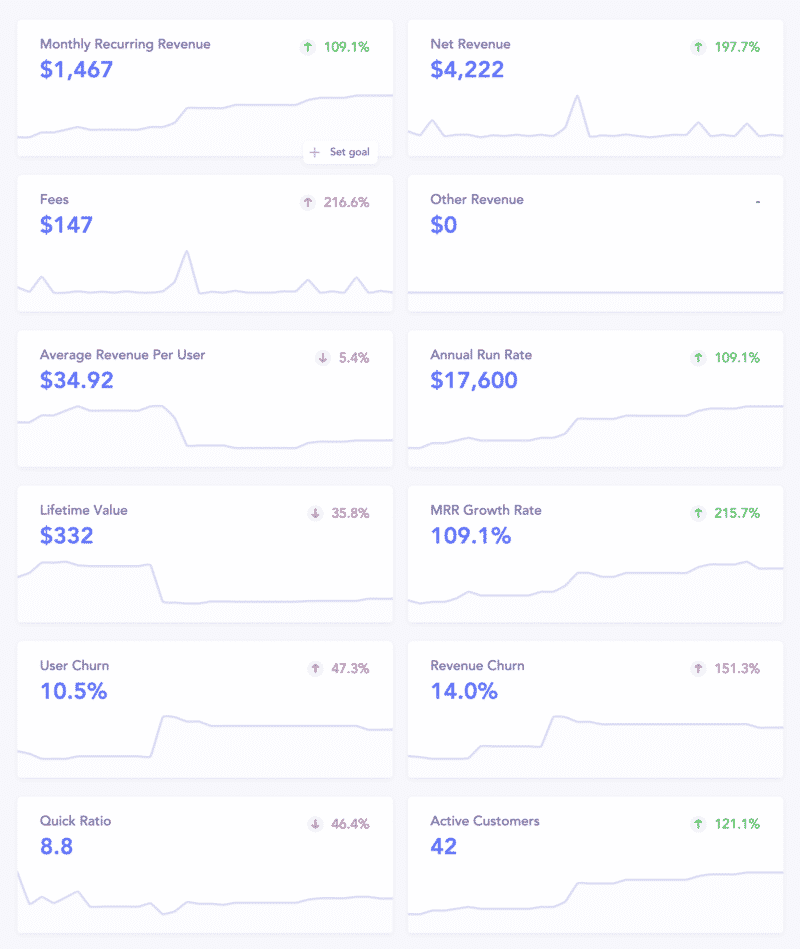**Detailed Caption:**

This image is a detailed screenshot of a financial dashboard, designed to track various business performance metrics. The dashboard occupies a space approximately five inches wide and eight inches tall, with a light blue outline. The interface is divided into 12 distinct boxes, each presenting a key financial indicator. 

At the top, there's a section labeled "Monthly Recurring Revenue," followed by metrics such as "Net Revenue," which likely represents the total income after expenses. Additionally, it includes fields for "Fees and Other Revenue," providing a breakdown of various income sources.

Prominently displayed metrics include "Average Revenue Per User" and the "Lifetime Value" of customers, which help gauge the long-term profitability of the business. The "Growth Rate," shown in blue at 109.1%, and another in green at 215.7%, likely differentiate between annual growth and total growth rates, indicating the business's expansion over time.

There is also a detail about "Active Customers," suggesting the dashboard can be used by businesses with recurring clientele, such as rental property owners or storage unit managers. Overall, this dashboard serves as a financial tool for small business owners, offering a consolidated view of revenue streams, profit margins, and growth trends.